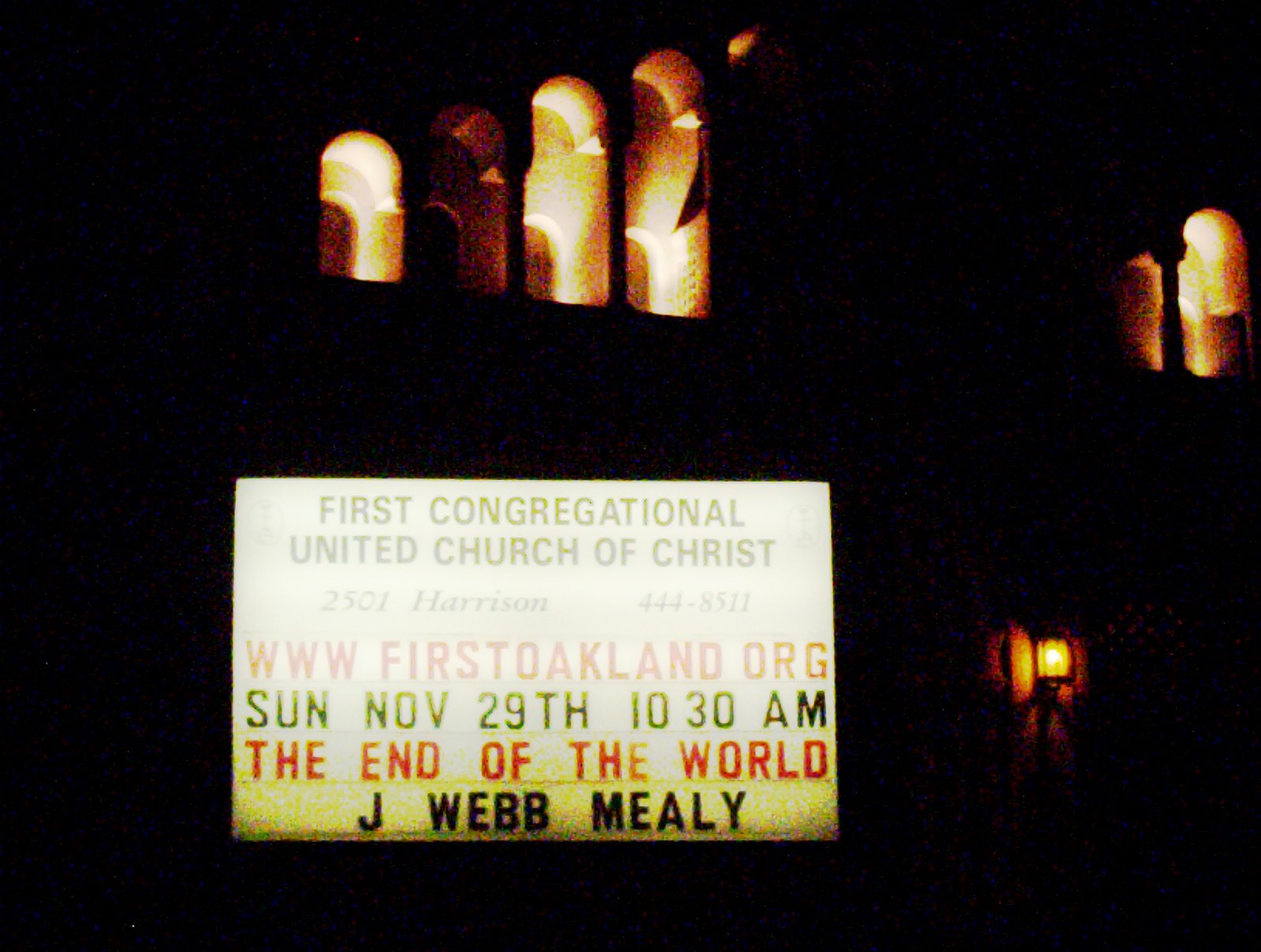This color photograph, taken at night in landscape orientation, captures the exterior of the First Congregational United Church of Christ. Dominating the bottom left of the image is a lit sign reminiscent of changeable church boards. The sign reads "First Congregational United Church of Christ" in black letters, and beneath it are the church's address, "2501 Harrison," and phone number, "444-8511," also in black. Below this, in red letters, is the website "www.firstoakland.org," notably without any dots separating the sections. Following this, the schedule "Sun, Nov 29th, 10:30 AM" is displayed in black letters. Another message in red beneath this announces "The End of the World," and in black text below, "J. Webb Mealy" is indicated.

The composition focuses on the glowing sign, contrasted by the dark surroundings. The church itself features arched openings on its second floor, which emit warm light, suggesting open windows without glass. There's also a small lantern on the right side, adding subtle illumination to the area near the church door. The style is a realistic representation of the scene, with emphasis on the illuminated elements against the night sky.